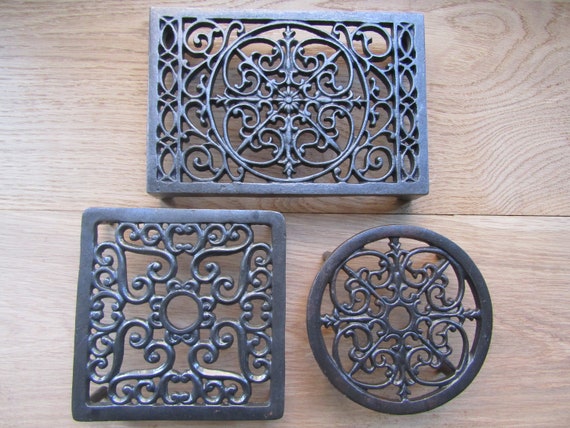On a rustic wooden table with visible slats, there are three ornate metal hot plate stands meticulously displayed. Each stand features an intricate doily-like design, evocative of the 1800s or early 1900s craftsmanship. The stands, varying in shape, consist of one rectangular, one square, and one circular piece. The rectangular stand, positioned at the back, showcases a unique iron pattern. Below it, to the left, the square stand is adorned with heart designs encircling a central motif. Adjacent to it on the right, the circular stand also incorporates heart shapes and a central design. All three stands are elevated on four small legs to ensure that hot pots do not scorch the table beneath. This elegant set of metal potholders is both functional and decorative, ideal for showcasing during a party or holiday gathering.